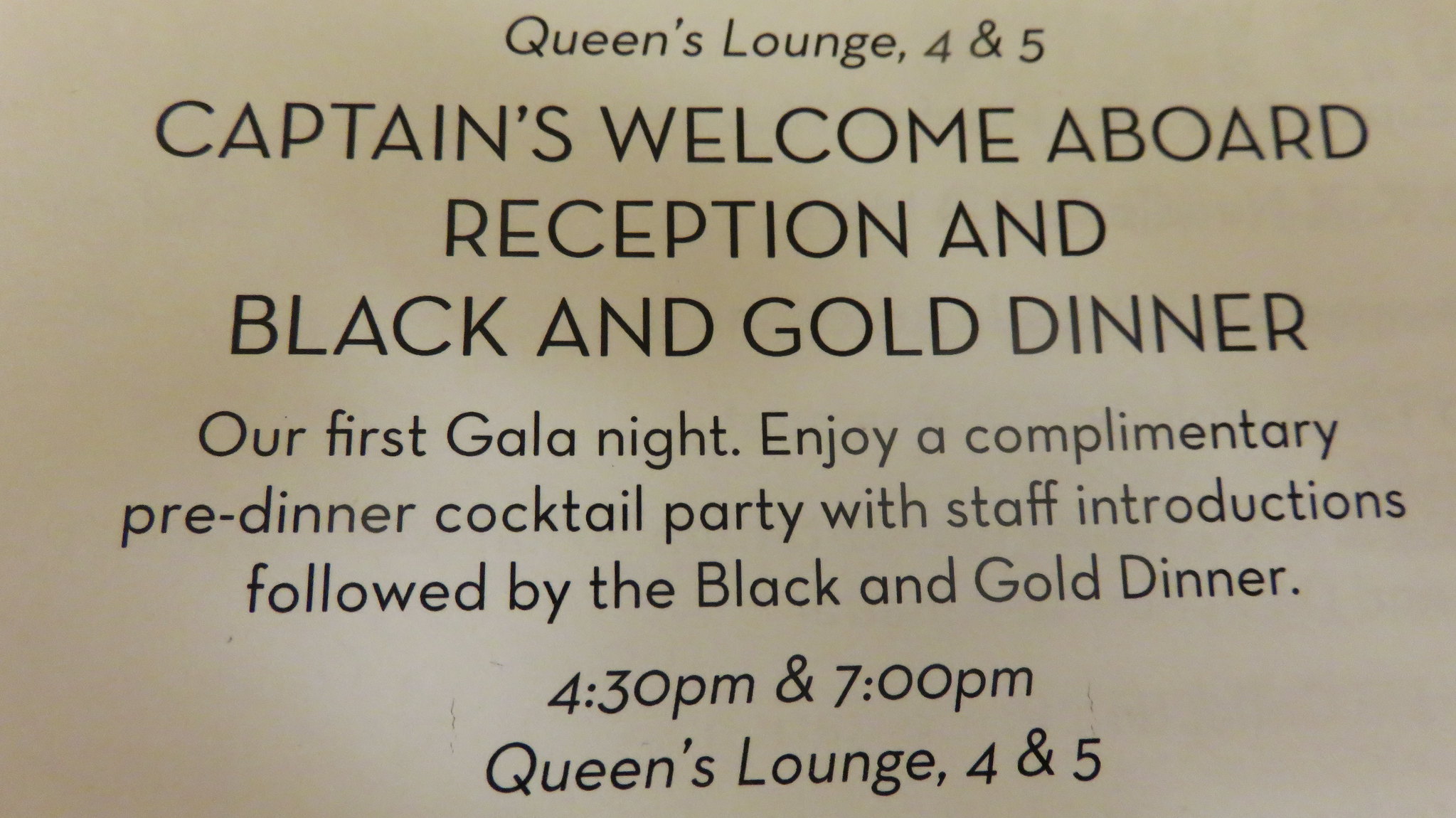This image features a simple advertisement with a grayish, tannish background and black centered text. At the top, it says "Queens Lounge, 4 and 5" in a smaller font with a capital "Q" and "L." Below this, in larger, bold, all-capital letters, it says "CAPTAIN'S WELCOME ABOARD, RECEPTION, AND BLACK AND GOLD DINNER." Following in standard text, the message reads: "Our first gala night. Enjoy a complimentary pre-dinner cocktail party with staff introductions, followed by the Black and Gold Dinner." The times for the event, "4:30 PM and 7:00 PM," are written in italics, with the final line reiterating "Queens Lounge, 4 and 5."